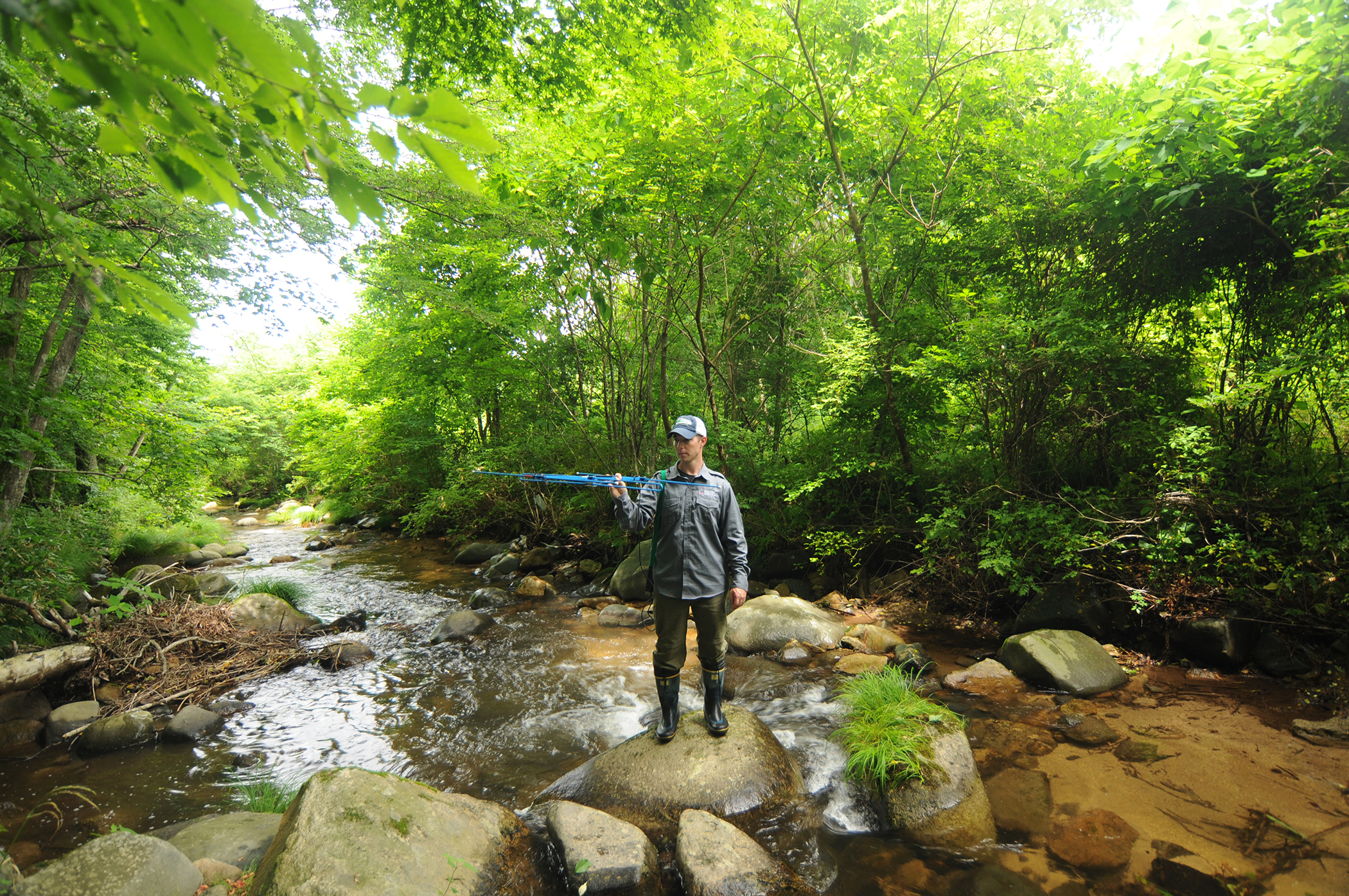In this serene forest setting, a man stands atop a large, wet, round rock in the middle of a freshwater stream, surrounded by lush, green trees. Sunlight filters through a tiny clearing in the foliage on the upper left, casting a gentle glow on the scene. The man, clad in a gray button-down shirt, olive trousers, and knee-high dark rubber boots, wears a baseball cap with a blue brim and a red and white back. His gaze is focused downwards, intently studying or measuring something with the blue stick-like instrument—possibly a fishing pole—in his right hand. The creek winds through the rocky landscape, with clusters of branches suggesting a potential beaver dam on one side. The peaceful backdrop of green trees and flowing water evokes a sense of quiet reflection and tranquility.